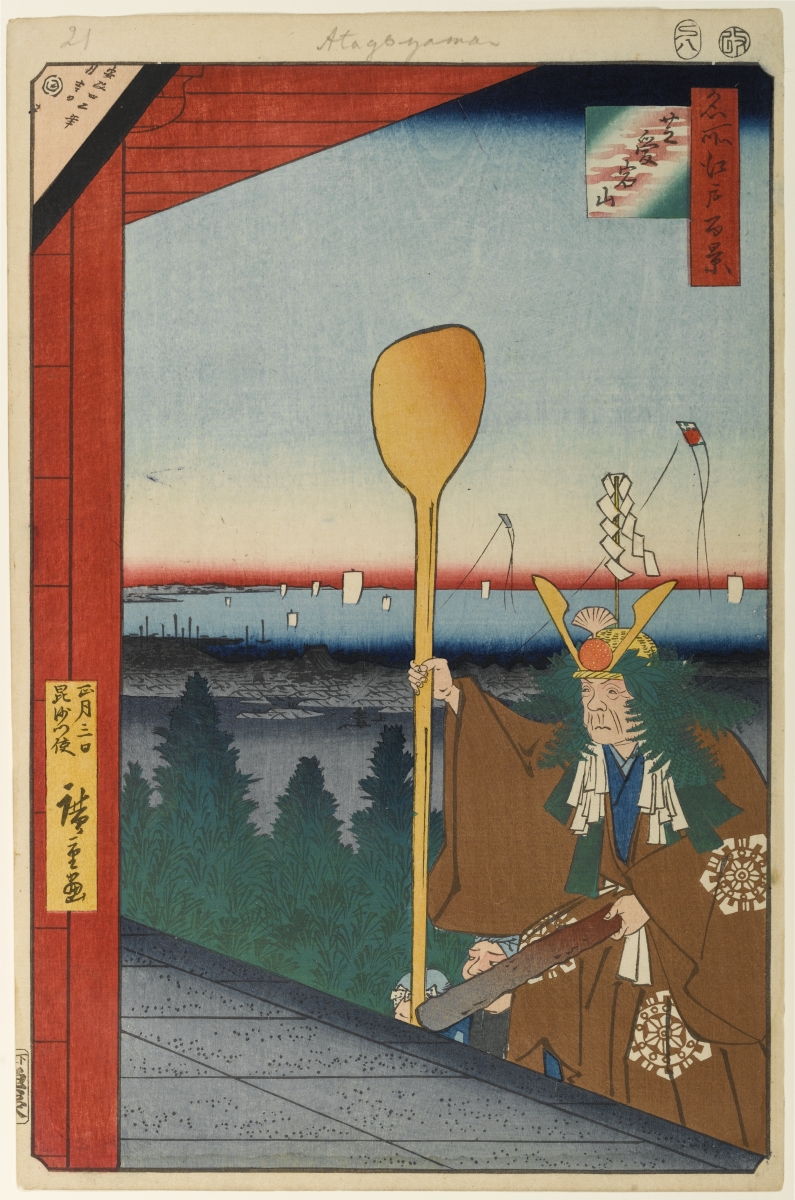This cartoon-like illustration, reminiscent of an ancient Japanese-style painting from the shogun periods, depicts a scene with water in the background, akin to a bog or a rice field, with white rectangular structures emerging from the water. The image is bordered on the left and top with a red trim that resembles a wooden door frame. In the bottom right corner, an elderly Oriental man is portrayed in a detailed manner. He is dressed in a large brown kimono-like robe adorned with cream-colored star or floral designs and a blue robe underneath. His headpiece is gold with green feathers or leaves sprouting from it, creating a striking visual effect akin to representing his hair. The old man, his face etched with wrinkles around his mouth, nose, and eyes, holds an oar or giant paddle in his right hand and a broad stick or club in his left. Behind him is an expanse of blue, possibly representing a lake or ocean, with some solitary sails visible. The composition is further enriched with Asian writing in the top left and along the left border, adding to the artwork's authentic cultural touch.